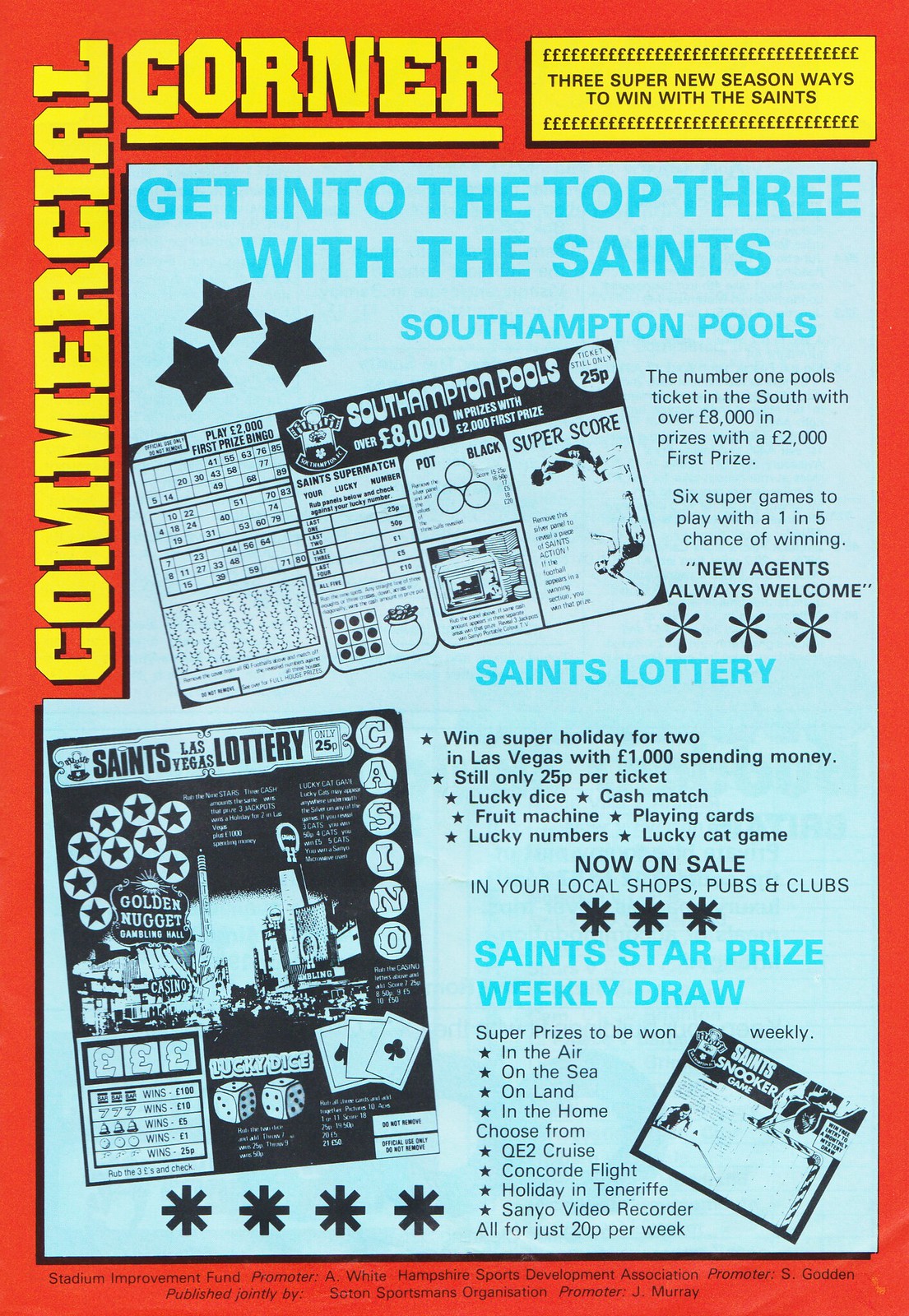This is a tall, vertical rectangular poster with a vibrant red background, possibly serving as a magazine cover or advertisement. Along the left edge, the word "COMMERCIAL" is written vertically in bold yellow uppercase letters. At the top of the poster, "CORNER" is written horizontally and underlined with a yellow line. In the upper right-hand corner, a yellow rectangle encloses black text that reads "Three super new season ways to win with the Saints."

Dominating the central area of the poster is a large white rectangle. At the top of this rectangle, blue print proclaims, "Get into the top three with the Saints." Below this headline, three black stars adorn the lower left area. Further down, the text promotes "Southampton Pools" with associated graphics resembling lottery tickets, which are black and white.

The middle section showcases the title "Saints Lottery" in blueprint, accompanied by star-shaped bullet points detailing various prize opportunities, including a super holiday for two and multiple ways to win for only $0.25 per ticket. The bottom section, headlined "Saints Star Prize Weekly Draw" in blue, lists additional prize details and emphasizes that the prize can be won weekly. The poster is vibrant and eye-catching, designed to attract attention with its structured and detailed layout.